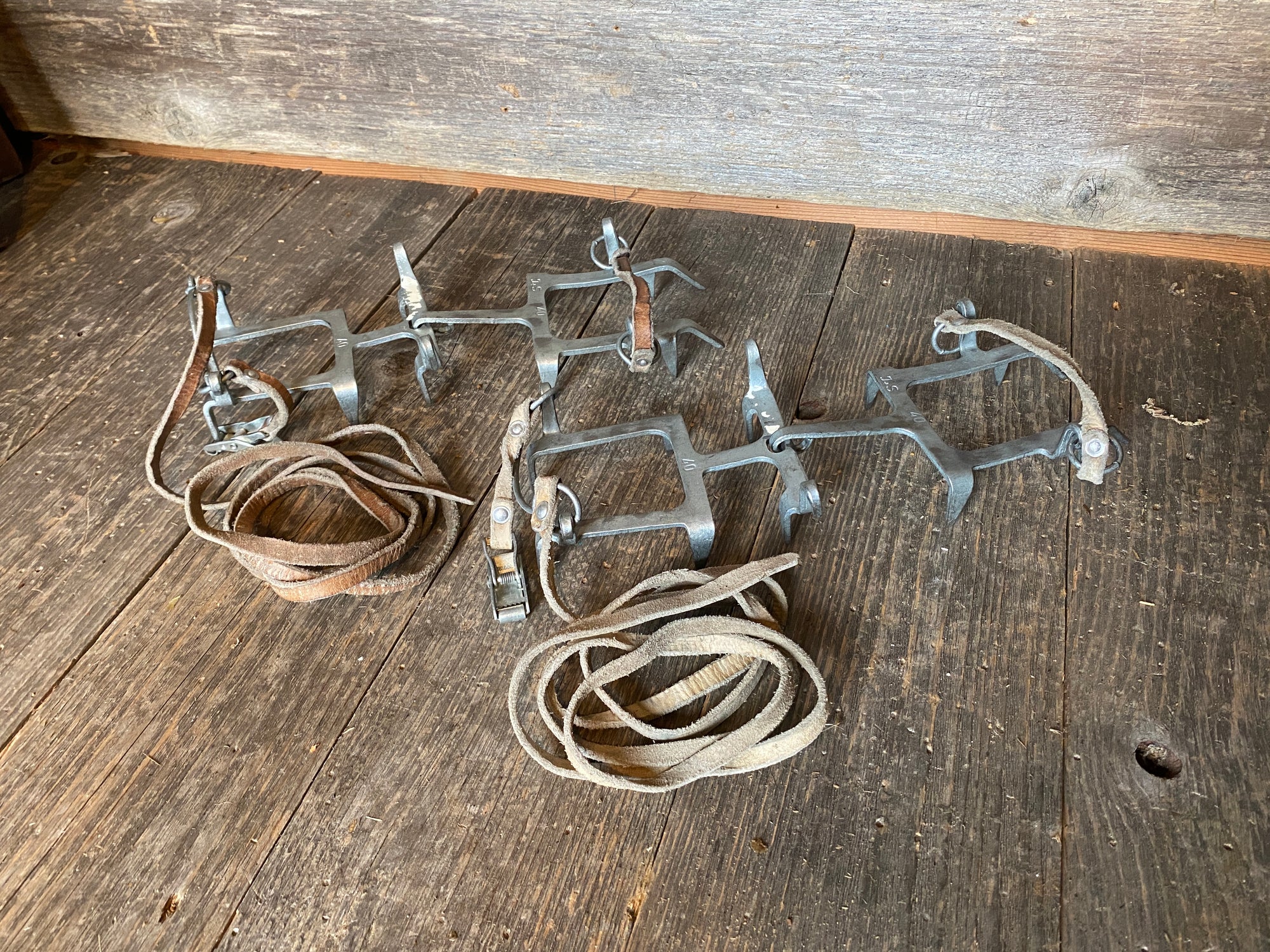In the image, a pair of vintage ice cleats, made of sturdy silver metal, are displayed on a rough, dark brown wooden floor, set against a light brown wooden wall. Each cleat consists of two interlocking, rectangular parts that hinge in the center and feature spikes at the corners. A worn leather strap, showing signs of wear and tear, is affixed to the bottom of each cleat, one with a lighter tan strap and the other with a darker brown strap. Despite their age, the metal components remain in good condition, evoking a sense of durability and historical craftsmanship. The scene is devoid of any text, allowing the viewer to appreciate the rustic and utilitarian aesthetic of these antique tools.